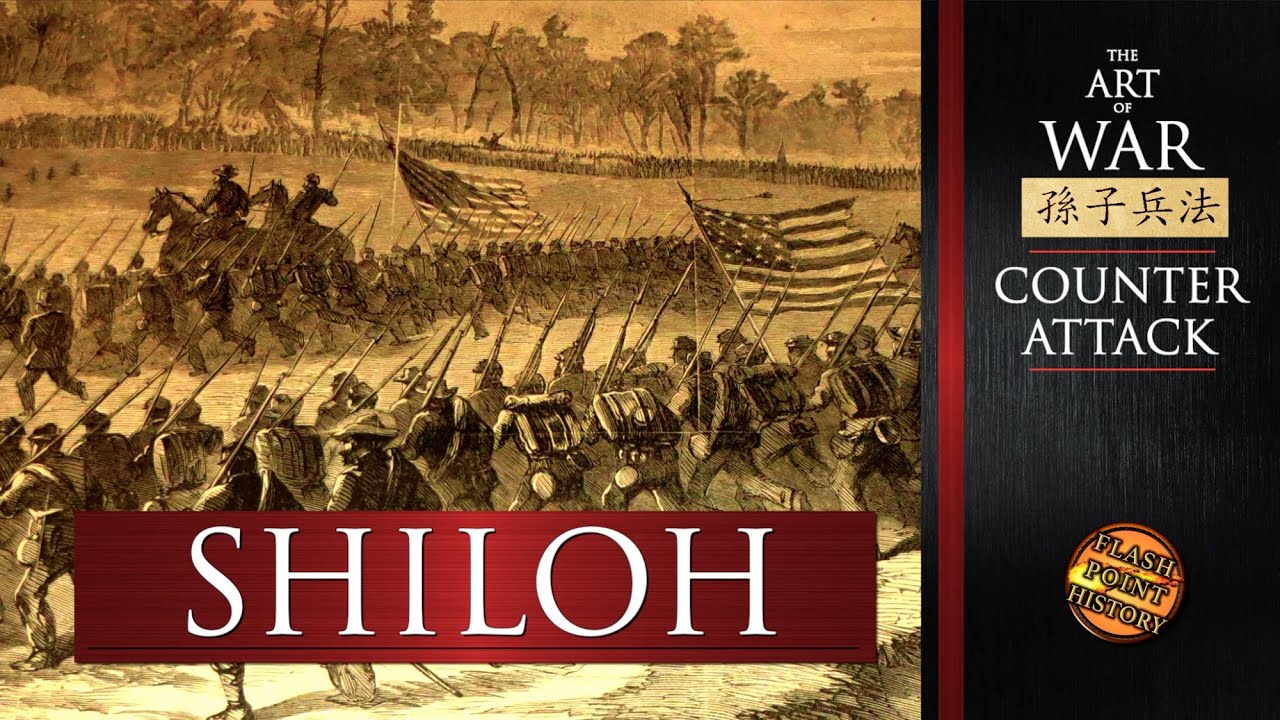The image, which resembles the cover of a book, is divided into two distinct sections. On the right side, there's a black vertical triangle with a red stripe on its left edge. At the top of this section, it says "The Art of War" with "The" in small writing, "Art" slightly larger, "of" very small, and "War" prominently displayed. Below this, there is some Asian script, possibly kanji, within a tan box, followed by "COUNTERATTACK" in all capital letters. Near the bottom of this section, a gold circle bears the inscription "Flashpoint History."

The left side of the cover depicts a historical battle scene, likely tied to the Battle of Shiloh from the American Civil War. The image includes an old brown depiction of that era, showing generals on horseback and troops advancing, with the American flag prominently displayed in two places. Text reading "Shiloh" in large white letters is set within a horizontal red rectangle at the bottom. The entire cover combines elements of historical military strategy and significant battle imagery.